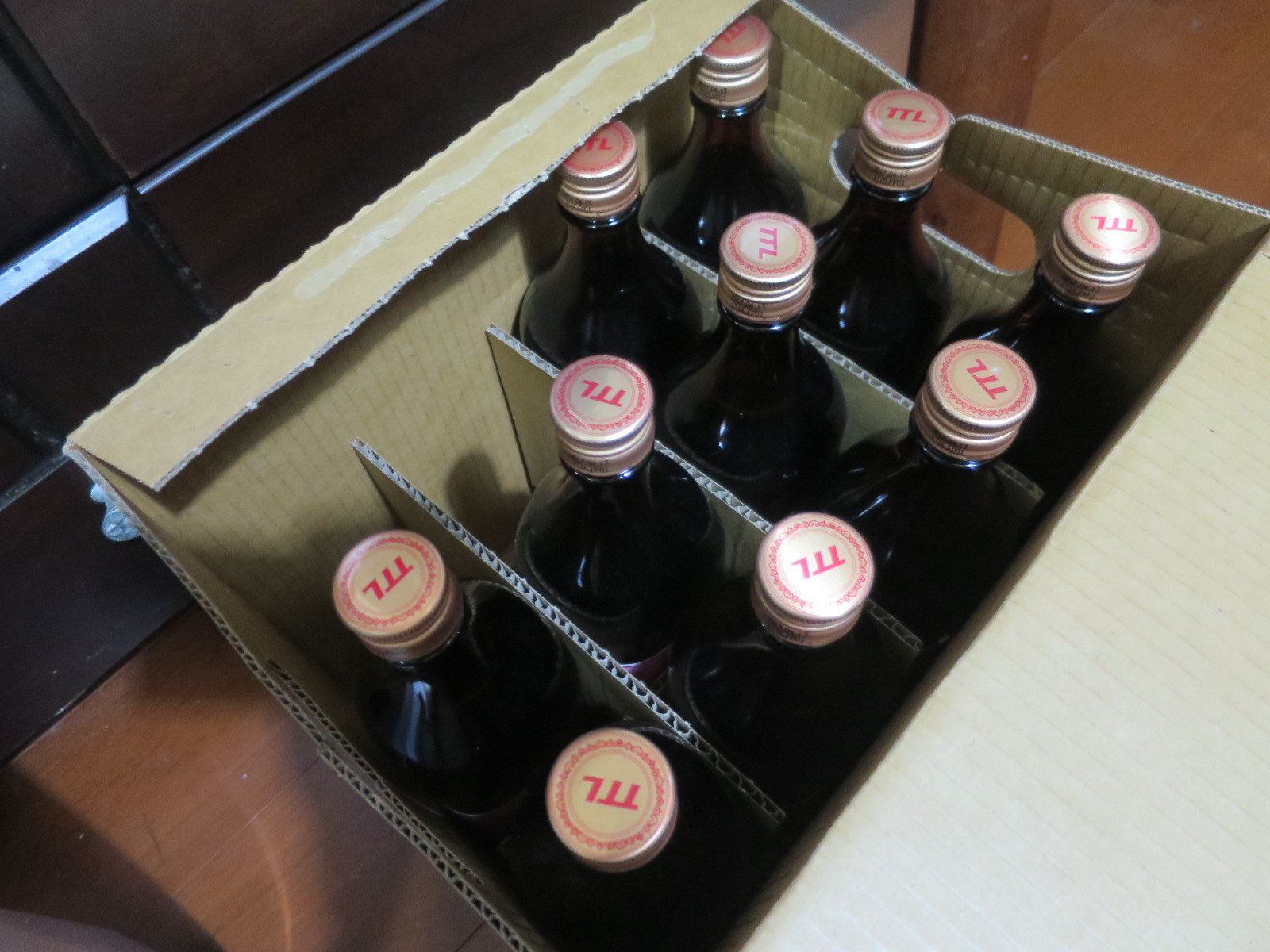This photograph captures a partially opened cardboard box designed to hold a dozen bottles, viewed from above and sitting on a wooden table, possibly in someone's home. The box, propped open with its lid hinged to the right, features cardboard partitions that create separate compartments for each bottle, ensuring they remain secure and protected during transport. Two of the bottles, specifically from the top left section of the box, have been removed, leaving only ten dark-colored bottles in the box. These bottles, possibly resembling olive oil or beer bottles, have silver twist-on caps adorned with a red emblem bearing the initials "TTL." In the blurred, darkened background, a bit of gleaming silver equipment, perhaps a refrigerator, can be seen. Overall, the image highlights the careful packaging and placement of the bottles, emphasizing their dark hue and distinctive cap design.